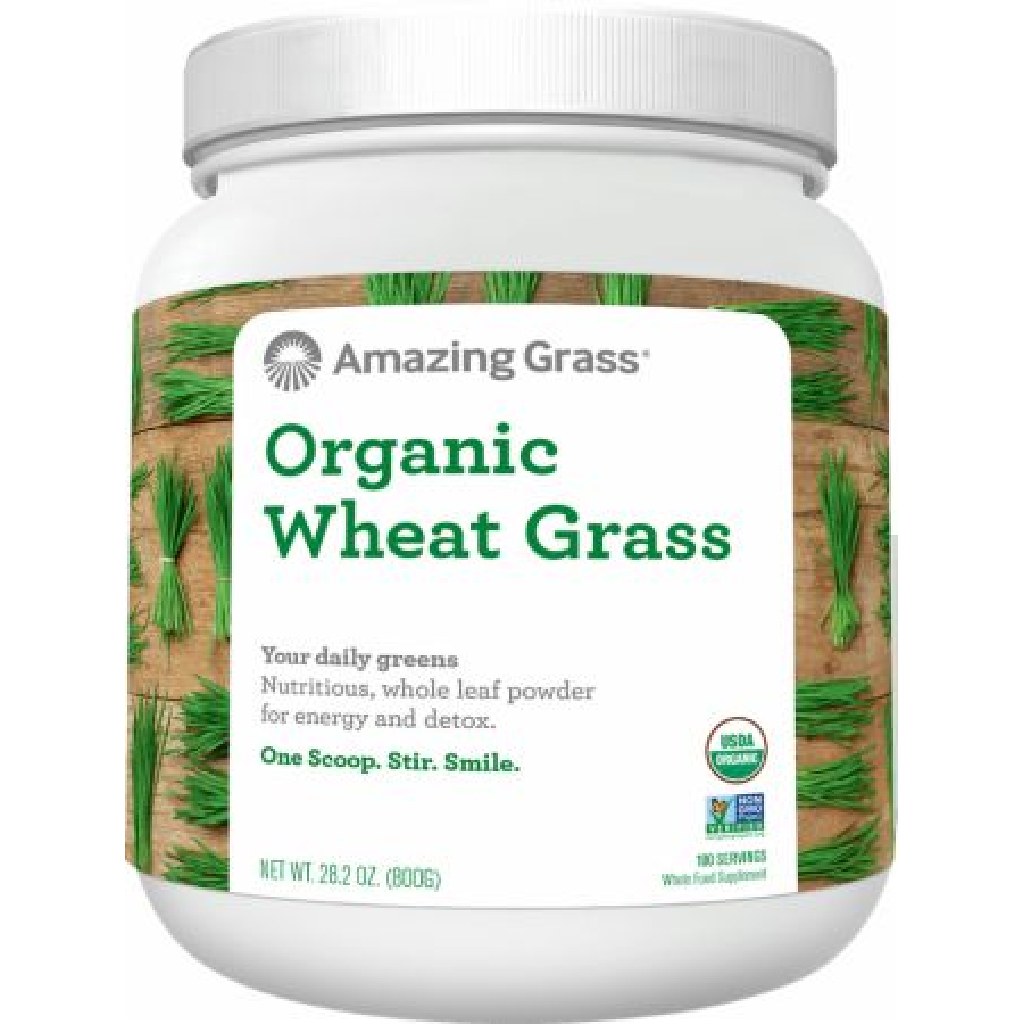The image captures a canister of organic wheat grass powder, prominently displayed against a backdrop of lush, green grass bunches set on a brown surface that could depict either a wooden fence or soil. Central to the image is a white label with clear, bold text reading "Organic Wheat Grass, Your Daily Greens." Additional instructions note, "One scoop, stir, smile," indicating its use as an ingredient for health shakes. The product has a net weight of 28.2 ounces, and in the bottom right-hand corner of the label, several certification logos are visible, attesting to its organic and health standards. The canister itself is white and is topped with a secure screw top lid. This product, while not commonly seen in this country, highlights the growing trend of integrating superfoods into daily diets.